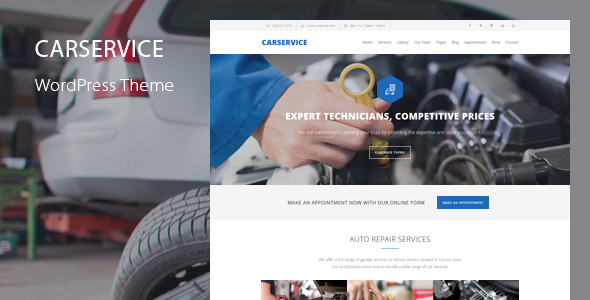The image showcases a WordPress theme titled "Car Service." In the preview, key elements include a header containing navigation links such as Home, Services, Gallery, Team, Blog, Appointment, and Contact. The central focus is a main image featuring a close-up of a mechanic's hands working on a car engine. Prominent text overlaying this image reads "Expert Technicians, Competitive Prices," followed by the subheading, "We are committed to earning your trust by providing the expertise and value you expect." A call-to-action button labeled "Make an Appointment" is also present, encouraging online form submissions for appointments.

Below the main image, there is a section titled "Auto Repair Services," which includes text highlighting the range of services offered. This section is accompanied by smaller images related to car repair activities, though these images are partially cut off. The overall design of the theme emphasizes professionalism and trust, targeting auto repair businesses seeking an online presence.

Additional tabs are visible within the image but are slightly blurry and difficult to make out. The design aims to convey a sense of reliability and expertise to potential customers.